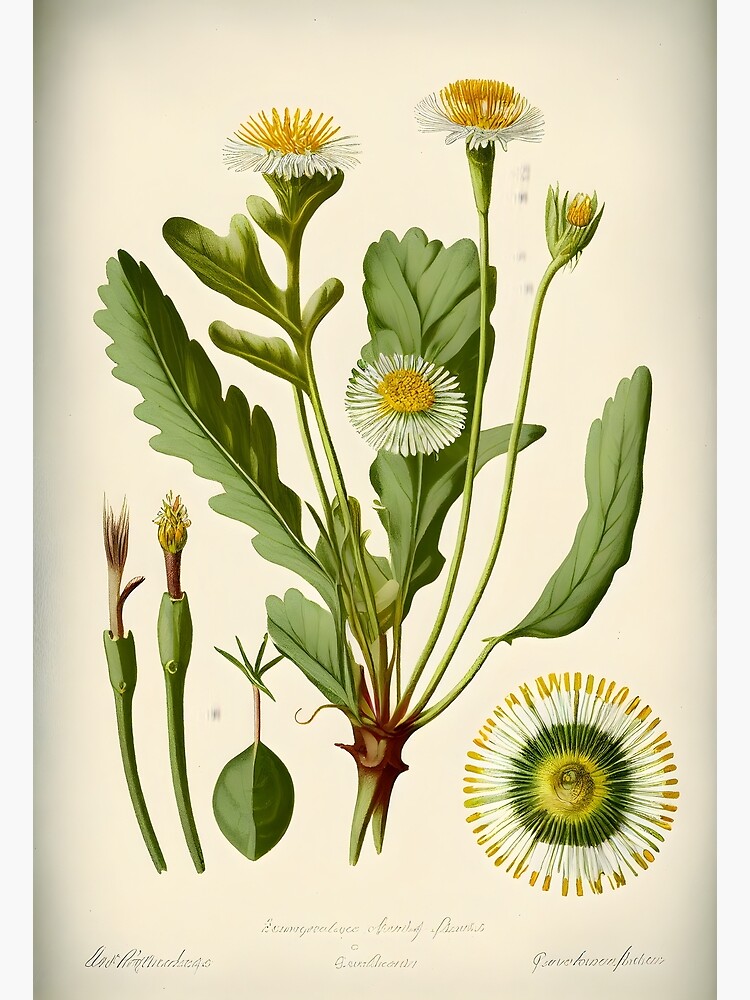This is a vintage-style hand-drawn illustration of a plant resembling a dandelion, set against a creamy beige background that darkens toward the edges. The primary focus is on three fully bloomed flowers with thin, white petals and yellow centers, showcasing intricate details such as the pistil, stamen, and anther. Surrounding these flowers are irregularly shaped, long green leaves and stems. To the left of the main image, there are diagrams showing the plant's stems and leaves, including several immature buds. On the right, there's a close-up of the flower's back and a more detailed view of a partially bloomed flower. At the bottom of the illustration, there is cursive writing that is hard to decipher, likely indicating the artist's name and title of the piece. The overall artwork has a rich color palette, adding to its detailed and botanical quality.